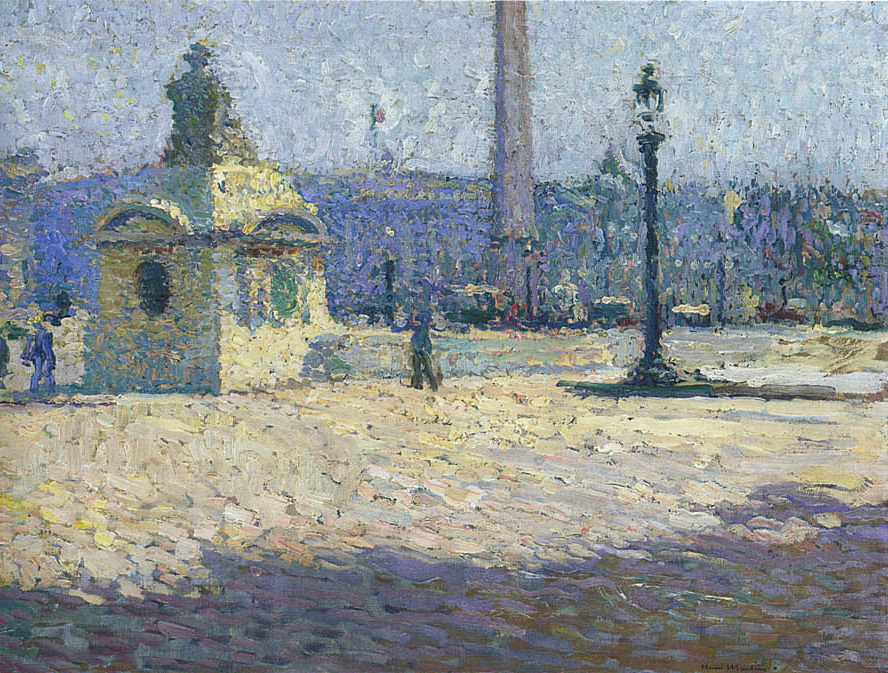The image is an oil painting depicting a bustling city square in the middle of the day. Dominating the left side of the image is a statue of a lady wearing a tall hat, which is perched atop a short building. The building features oval windows on all visible sides, each topped with an arched shape. Adjacent to the statue, on the right, is a short flight of stairs leading to the ground level. To the right of the stairs stands a tall, black lamppost. The square itself is populated with a few people walking around, including one person centered in the middle of the image. The ground is painted in a vibrant yellow, contrasting with the various colors used throughout the scene, such as lavender, gray, black, tan, orange, red, purple, pink, white, and yellow. The top of the image captures a portion of the sky, adding to the outdoor setting. Overall, the painting combines detailed architectural elements and human presence, creating a lively urban atmosphere.